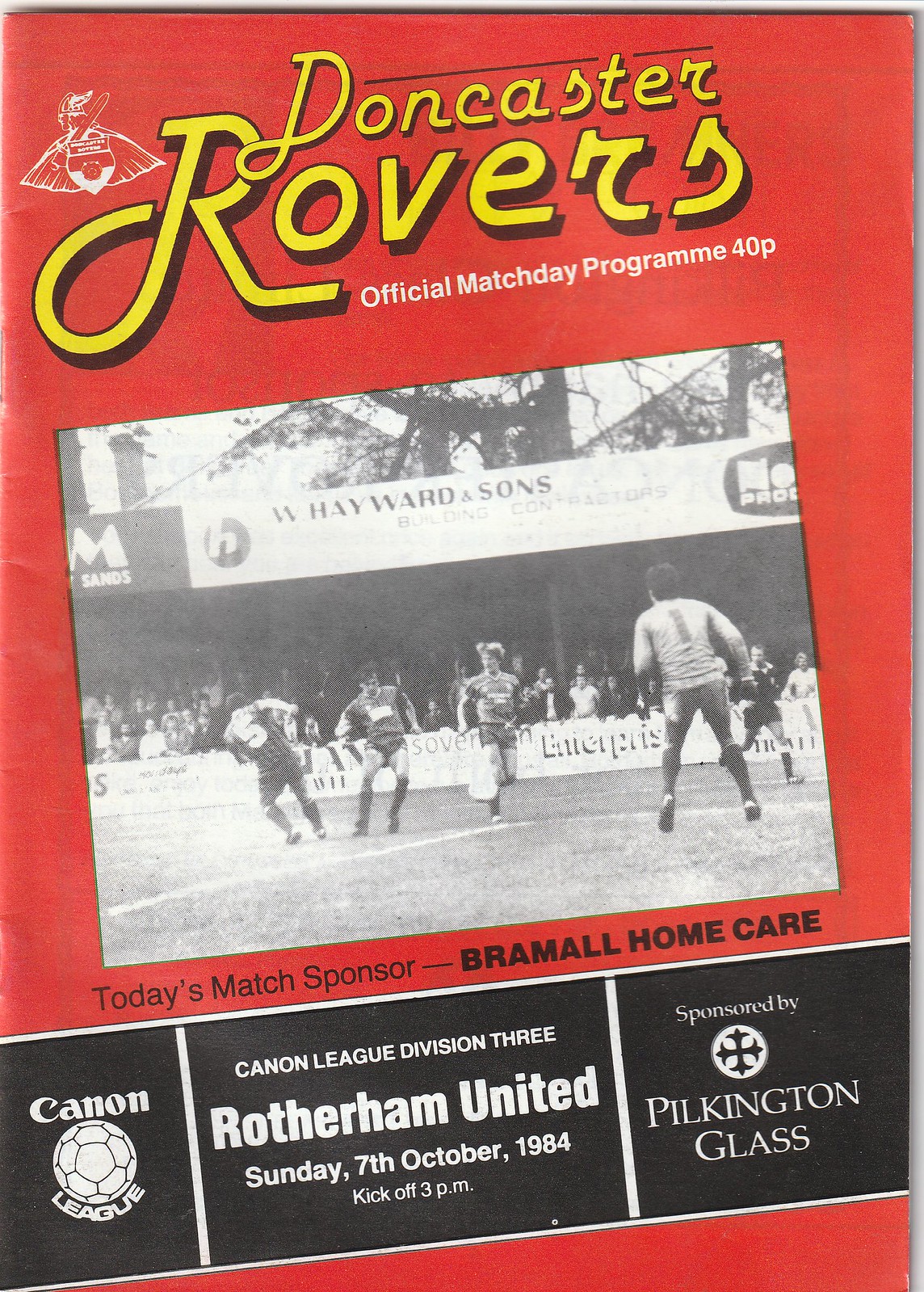The cover of the Doncaster Rovers Official Match Day Program from October 7, 1984, features a striking red background. At the top, prominently displayed in large yellow text, is the title "Doncaster Rovers," with the "R" notably larger than the other letters, outlined in black. Just beneath this, in white text, it reads "Official Match Day Program 40P." To the left of the title is the team's emblem—a white knight with a cape, holding a sword beside a shield.

Central to the cover is a black-and-white photograph showing a dynamic scene from a soccer match featuring four players prominently in the foreground, with more players and an enthusiastic crowd visible in the background. Behind the crowd are signs, one of which reads "W. Hayward and Sons" on a white background with black text. Trees can be seen lining the top background of the image.

Below the photograph, additional text in black font announces: "Today's Match Sponsor, Bramall Home Care." The bottom section of the cover is a black banner featuring three elements: on the left, "Canon League," with a soccer ball icon; in the center, "Canon League Division III, Rotherham United, Sunday, 7th October 1984, kickoff 3pm"; and on the right, "Sponsored by Pilkington Glass," with their logo—a white circle featuring a black cross.